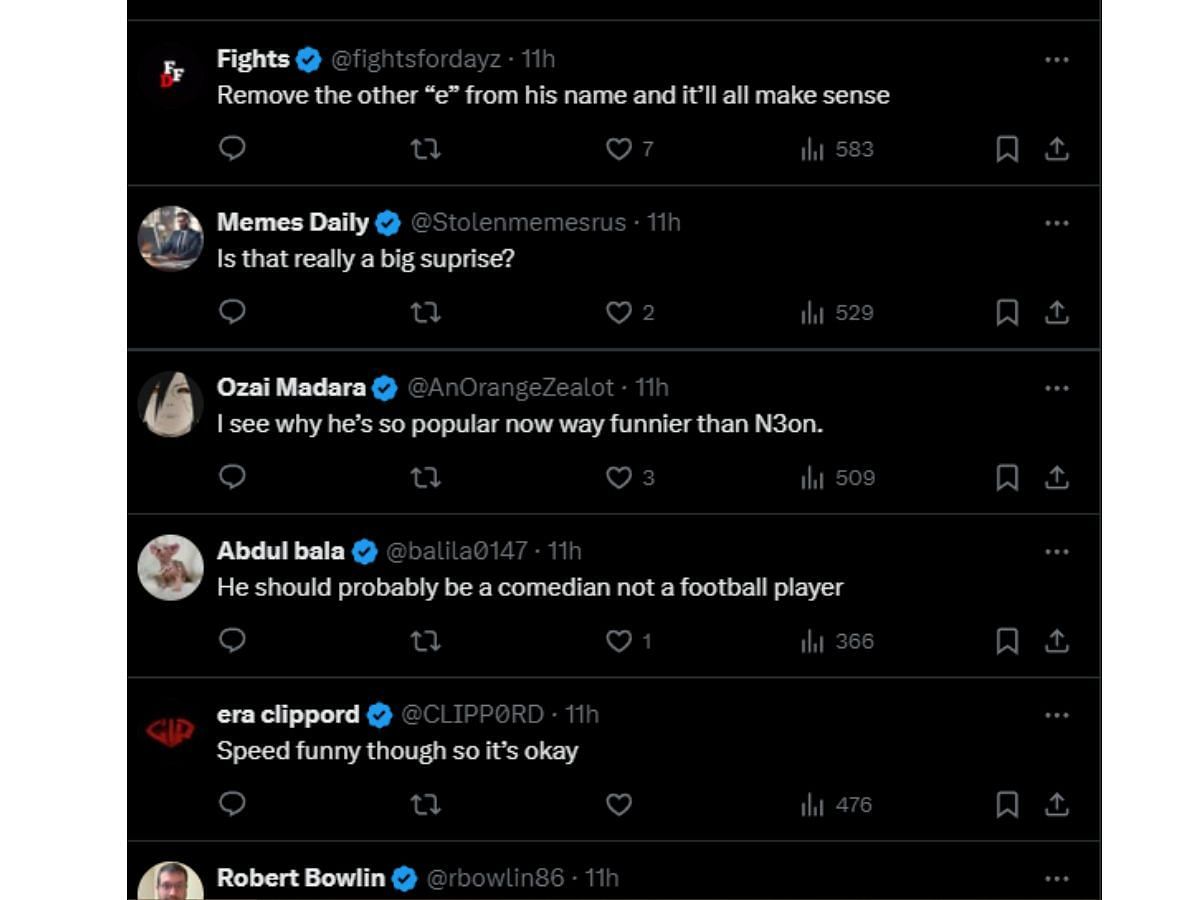The image has a predominantly black background. In the upper left-hand corner, there is an icon, followed by the bold text "FIGHTS." To the right, a blue certificate emblem with a black check mark reads, "AT FIGHTS FOR DAYS," ending with a stylized "Z," followed by "⋅ 11H." Adjacent to this are three horizontal light gray dots. Below this text, another line reads, "REMOVE THE OTHER (E) FROM HIS NAME, AND IT'LL MAKE SENSE."

Further down, there are several icons: a speech bubble, rotating arrows in a square shape, a heart with the number "7," a stats icon showing "583," a bookmark symbol, and an arrow pointing up over a bent line.

Below that, a circular icon shows "MEMES DAILY" in bold, accompanied by a similar certificate shape and check mark, noted with "AT STOLEN MEMESAURUS ⋅ 11 hours." Beneath this, the text reads, "IS THAT REALLY A BIG SURPRISE?" Following this, more icons appear: a speech bubble, a square in a circular shape, a heart displaying "529," a stats icon, a bookmark symbol, and an arrow pointing up.